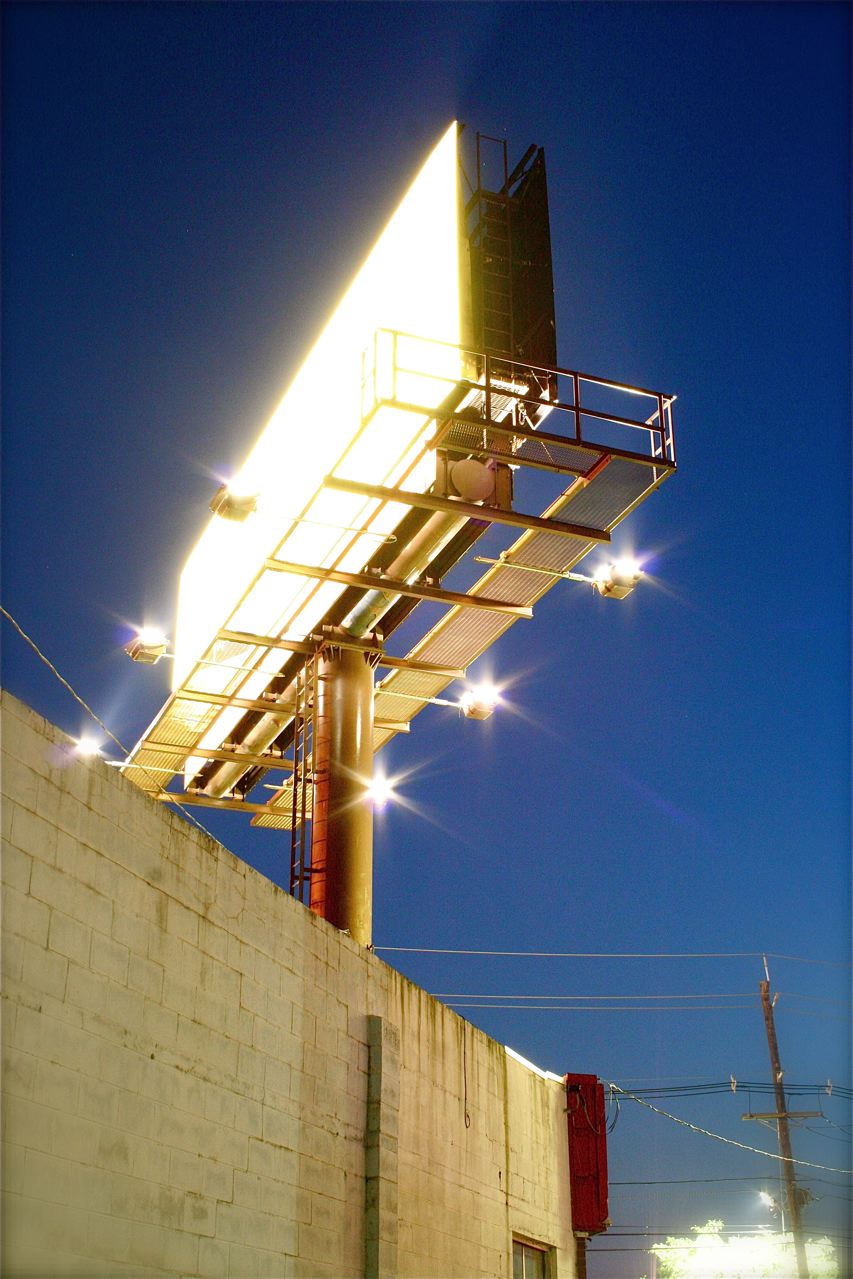In the overexposed nighttime scene, we gaze upward from the ground at a luminous billboard, its light intensely starburst and saturated in brightness. The beams from floodlights positioned on either side of the billboard cast additional light upwards, making the entire structure glow with overbearing brilliance. The billboard itself, a radiant rectangle, is so intensely illuminated that its contents are indiscernible, shrouded in a wash of white light.

Supporting this glowing display is a thick, round column, steadfast and sturdy, with a ladder affixed to it, leading to an access platform on either side of the billboard, hinting at maintenance and function in an otherwise stark composition. The entire structure stands atop a low cinder block wall, its coarse texture contrasting with the polished smoothness of the column.

In the background, more overexposed lights punctuate the dark, sprawling scene, forming clusters of starred glows against the night. Power lines crisscross the upper portions of the image, silhouetted against the artificial luminosity, adding an element of industrial complexity to this night-lit tableau.